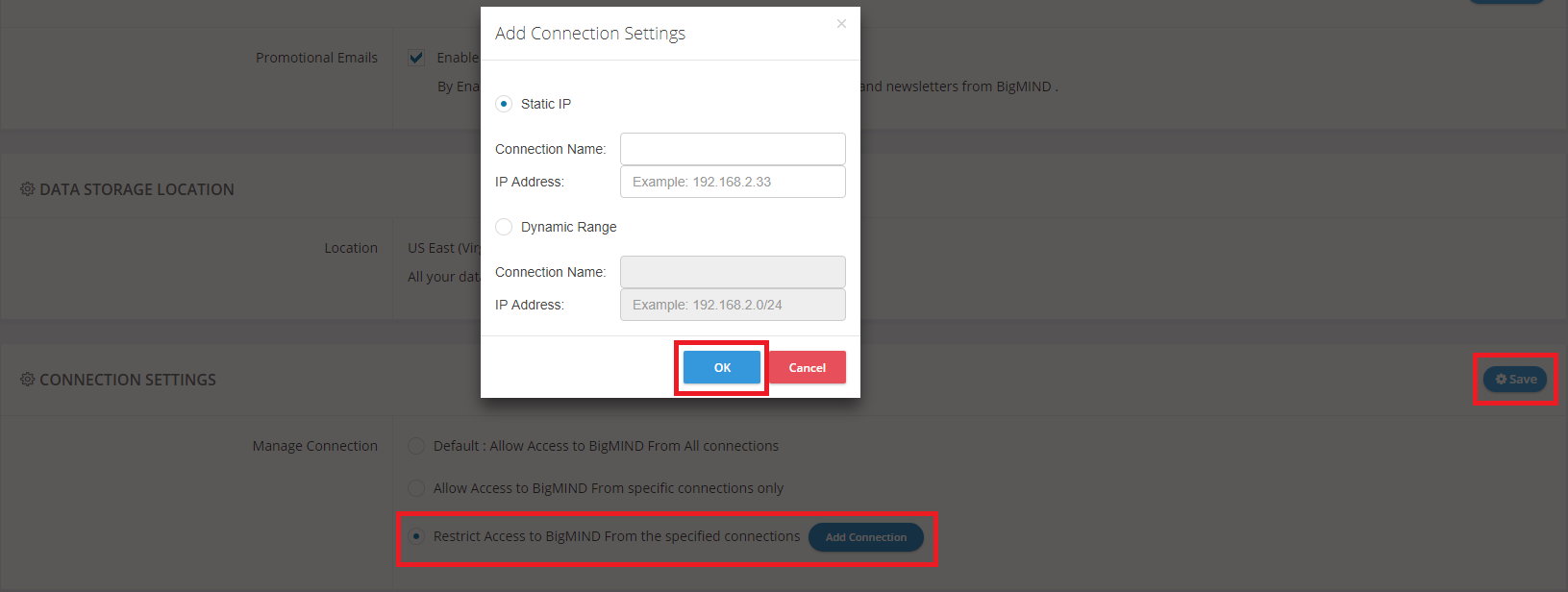This image is a detailed screenshot of a settings interface within a website or application. The background is grayed out by a translucent overlay, ensuring that the primary focus is on the settings panel in the foreground. The settings interface is divided into three primary sections.

At the very top, the interface title "Add Connection Settings" is displayed on a white background. Immediately beneath this title, the first setting labeled "Static IP" is selected, indicated by a highlighted toggle on the left. Below this, there is an input field for entering a "Connection Name" alongside a box on the right side for entering the desired name. Beneath this field, there is another section for entering an "IP Address," which is currently blank.

The remaining parts of the interface are slightly blurred but still partially legible. On the left side of the screen, the label "Data Storage Location" appears, followed by a section labeled "Connection Settings." At the bottom, an outlined area in red contains the text "Restrict access to Big Mind from specified connections." To the right of this text, there is a prominent blue button labeled "Add Connections." Multiple circles, presumably toggles for different connection settings, are displayed on the left side of this section, with one of them currently selected.